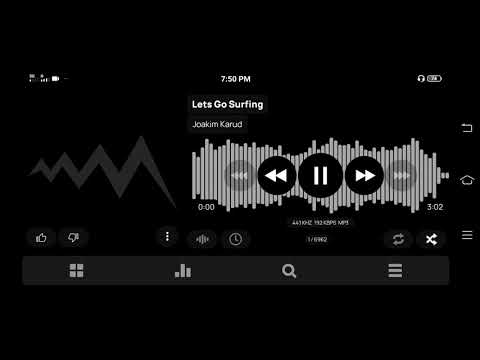The image features a sleek, black background with a digital music interface displayed prominently. At the center, in bold white text, the time is shown as "7:50 PM." On the right side near the time, a small headphone icon is visible, along with a battery life indicator, suggesting the listener is using a portable device.

Beneath the time, the text "Let's Go Surfing" is displayed in white, indicating the current song title. Directly underneath, the artist's name, "Joakim Karud," is clearly spelled out.

Stretching across the image are several horizontal white bars of varying lengths, representing a visual timeline of the song's progress. The song starts at "0:00" on the left and ends at "3:02" on the right. Positioned along these bars are three black circles: the left circle contains a white left-pointing arrow (indicating a previous track or rewind function), the middle circle features two vertical white lines (representing pause/play functionality), and the right circle shows a white right-pointing arrow (indicating next track or fast forward).

Towards the bottom of the interface, on the left, there are thumbs-up and thumbs-down icons, likely for rating the song. On the right, there's a pair of intersecting arrows (possibly for shuffle or repeat functions) and a three-bar icon, which might be used for accessing a menu or additional options.